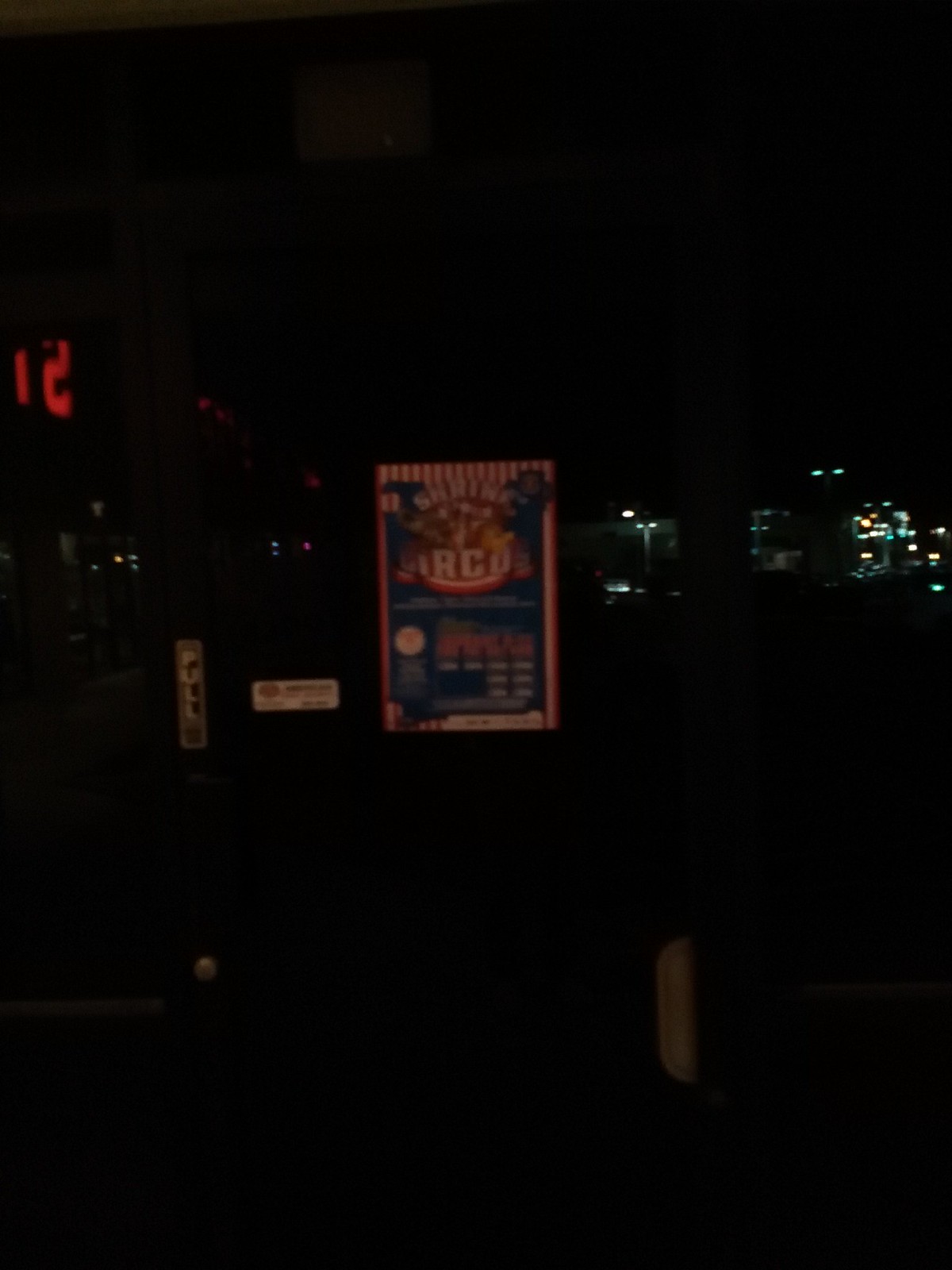This image is characterized by its low quality and resolution, appearing blurry, dark, and fuzzy. The majority of the image is engulfed in pitch-black darkness, with minimal discernable elements. At the center of the image, a rectangular poster is faintly visible. This poster predominantly features blue, red, and white hues. Although the text on the poster is illegible due to the blurriness, its presence is still noticeable. On the bottom left corner of the poster, a white sticker can be discerned. Additionally, to the left of the poster, there is another sticker with the word "PULL" in white text.